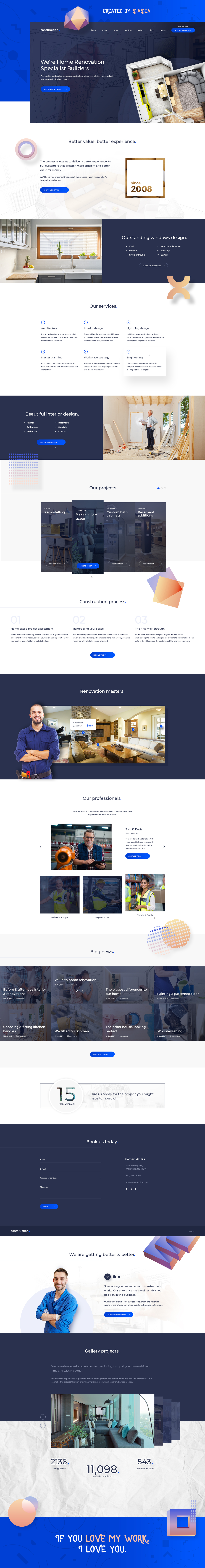This is an image of a home renovation website. At the top of the page, bold text announces, "We're Home Renovation Specialist Builders." Below this, the site highlights its establishment year, "2008," and promotes its value proposition with the phrase, "Better Value, Better Experience." The central portion of the image features a sleek kitchen showcasing a white counter and silver sink, adorned with a plate holding a pineapple and a plant sitting on the windowsill. Additional text emphasizes the company's focus on exquisite living spaces with the line, "Beautiful Interior Design." Also featured is a photograph of a smiling man in his early thirties, dressed in a blue work uniform and a tool belt filled with tools, suggesting his hands-on expertise in renovations. The bottom of the page contains a personal touch with the text, "If you love my work, I love you." The overall layout includes several tiny screenshots of different sections of the website, hinting at a comprehensive range of services and projects showcased on the site.